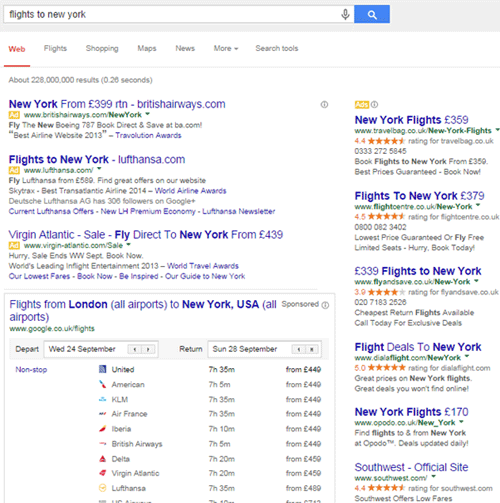The image showcases a Google search results page for the query "flight to New York." The search bar at the top clearly displays this query. The search results are categorized by titles in blue, URLs in green, and descriptions in black. 

1. The first result is titled "New York from £399 right now" from britishairways.com. The URL is britishairways.com, and the description reads: "Fly the new Boeing 787. Book direct and save at book.com. Best Airline Website Travel Solution Award."
2. The second result is from loothunter.com, titled "Flight to New York." It mentions a sale from Virgin Atlantic with direct flights to New York starting at £499. The URL is virginatlantic.com.

At the bottom, there is a list titled "Flight from London (All Airports) to New York, USA (All Airports)." The URL for this list is google.co.uk. The list details several flight options:

- Departing Wednesday, 24th September and returning Sunday, 28th September.
- Non-stop flights include: 
  - United, from £407, taking 7 hours 35 minutes.
  - American Airlines, from £440, taking 7 hours 5 minutes.
  - KLM, from £440.
  - Air France, same price as KLM.
  - Liberia Airlines, same price as KLM.
  - British Airways, same price as KLM.
  - Delta Airlines at £459.
  - Virgin Atlantic, same price as Delta.
  - Loothunter at £489.
  
The prices are listed on the right side in black. Additionally, on the right side of the page, there are various ads promoting New York flights, including:

- New York flights starting at £359 from flightcenter.co.uk, flightandsave.co.uk, delta-flights, airport.co.uk, and southwest.